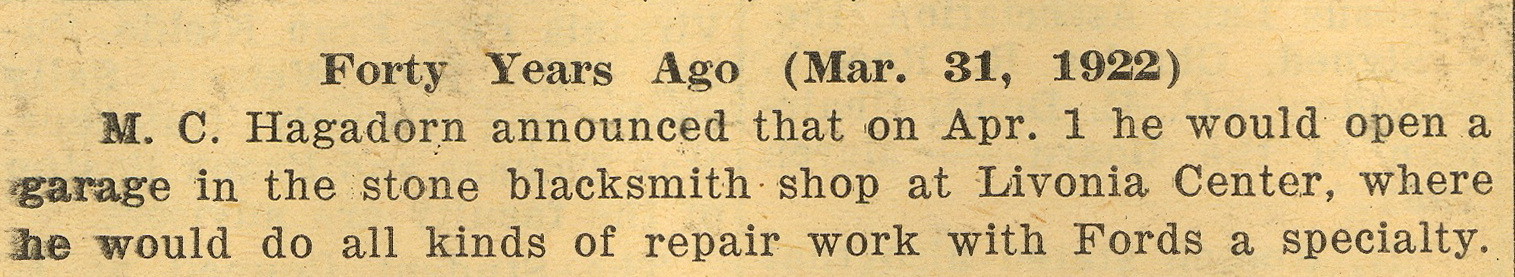This image depicts a yellowed, vintage newspaper clipping with a distinctly aged appearance, its cream-colored paper revealing its historical nature. The headline, boldly printed in an old-style font, reads "40 years ago, March 31st, 1922." Below, it describes M.C. Hagedorn's announcement of his new garage opening on April 1st at the Stone Blacksmith Shop in Livonia Center, specializing in all kinds of repair work, particularly for Ford vehicles. Despite some smudges and the slightly translucent paper hinting at text on the reverse side, the clipping remains untorn with surprisingly crisp edges.